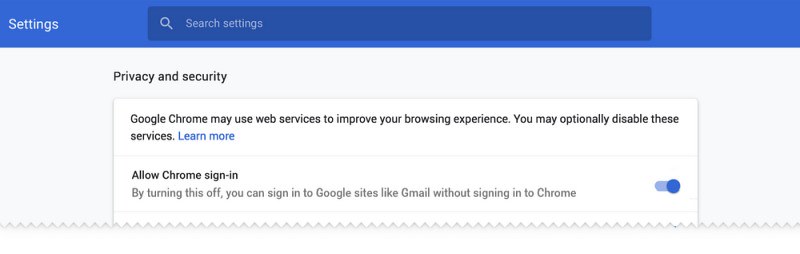The image captures a segment of a computer screen displaying the settings interface. The top of the interface features a narrow, blue bar. On the left side of this blue bar, the word "Settings" appears in white text. Centrally located beneath the blue bar is a search box, accompanied by a magnifying glass icon and the prompt "Search settings."

In the white section below, the heading "Privacy and security" is prominently displayed in black text. Midway down, a white box contains a message in black text that reads: "Google Chrome may use web services to improve your browsing experience. You may optionally disable these services." Under this text, a "Learn more" link is highlighted in blue.

Further down, there is an option labeled "Allow Chrome sign-in" in black text. Directly beneath this, gray text clarifies, "By turning this off, you can sign into Google sites like Gmail without signing into Chrome." Adjacent to this explanation is a small blue toggle button, allowing users to switch the setting on or off.

The bottom portion of the image appears cut off, with a jagged, uneven edge resembling the pattern created by pinking shears, hinting that the screenshot is incomplete. Overall, the image presents a detailed view of Google Chrome's privacy and security settings interface.